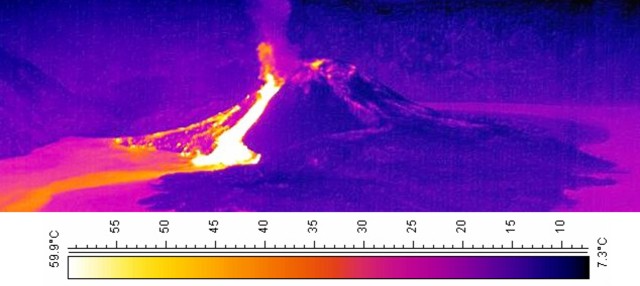The image depicts a thermal imaging view of a semi-erupting volcano set against a strikingly colorful background. At the center of the rectangular and horizontally elongated photo, the volcano releases a mixture of vibrant hues, including orange and yellow magma spilling down its left side, intermingled with light purple and pink smoke escaping from its base. The sky behind the volcano transitions through various deep shades of purple, indigo, navy blue, and black.

A notable feature in the image is a temperature scale bar along the bottom edge, which measures the temperature in degrees Celsius, ranging from 7.3°C on the right to 59.9°C on the left, with increments marked every 5 degrees. The colors of the scale follow a gradient from white, representing the hottest areas, to yellow, orange, red, pink, purple, blue, and finally black, indicating the coolest temperatures. This scale, alongside the thermal imaging, conveys the varying heat intensities within the scene, enhancing the dynamic and vivid presentation of the erupting volcano.